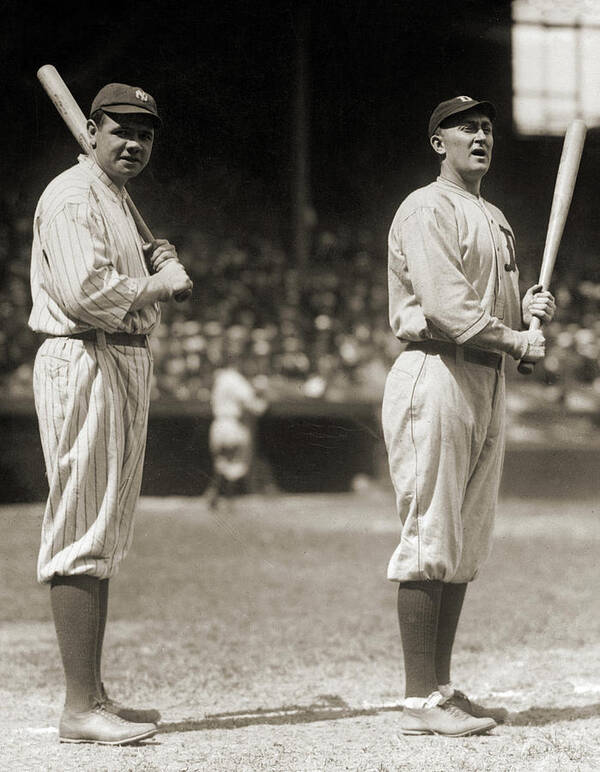This black-and-white photograph, likely taken in the 1920s or 1930s, captures two legendary baseball players on a professional field. The player on the left is Babe Ruth, donned in a classic New York Yankees uniform with pinstripes. Ruth's outfit includes a dark Yankees cap, a pinstriped shirt, white pants with black stripes, and dark stockings tucked into what appear to be dress shoes. He stands facing the right side of the image but turns his head to gaze directly into the camera, holding a bat over his left shoulder.

To his right stands another iconic player, Ty Cobb, in a Detroit Tigers uniform. Cobb is dressed in plain white attire with a dark belt and socks. His cap features the Old English “D” of Detroit, matching the letter inscribed on his chest. Unlike Ruth, Cobb is looking off into the distance with his mouth slightly open, holding his bat in both hands in front of him.

Both players are casting shadows on the dirt field, standing in the foreground with a blurred background that hints at a crowded stadium. The indistinct figures in the stands and an additional blurry player contribute to the nostalgic ambiance of this historic image.